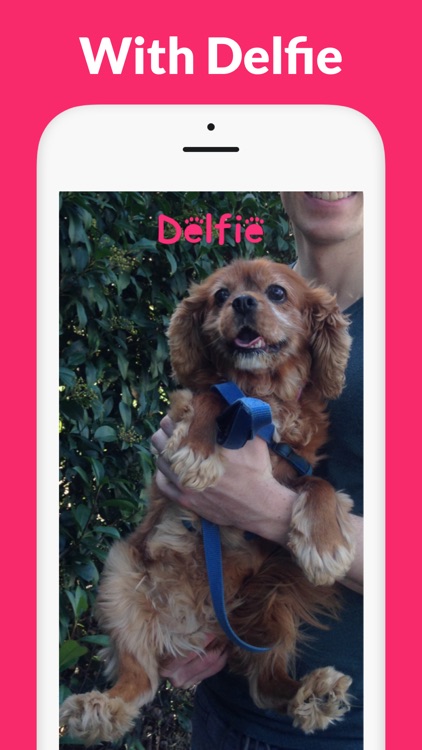The image features a predominantly pink, nearly square background with large, centrally placed white font displaying the text "Delphi." The text is complemented by a white-outlined illustration of a cell phone, which contains a photo of a light and dark brown dog with black eyes and a black nose. This endearing dog, named Delphi, proudly wears a blue collar and leash.

Inside the white-outlined cell phone, the dog's image is centered with a black dot and line highlighting specific details. The dog's name, "Delphi," is emblazoned in white with paw print accents above the second and last 'E'. The dog has light brown fur on its inner areas and darker, thicker fur on the outer parts.

A white Caucasian person, dressed in a dark top, is holding the dog from underneath its paws. The person's hand supports the dog, who gazes upward with a joyful expression, displaying a big smile. The background behind the dog is subtly decorated with green leaves, adding a touch of natural beauty to the portrait.